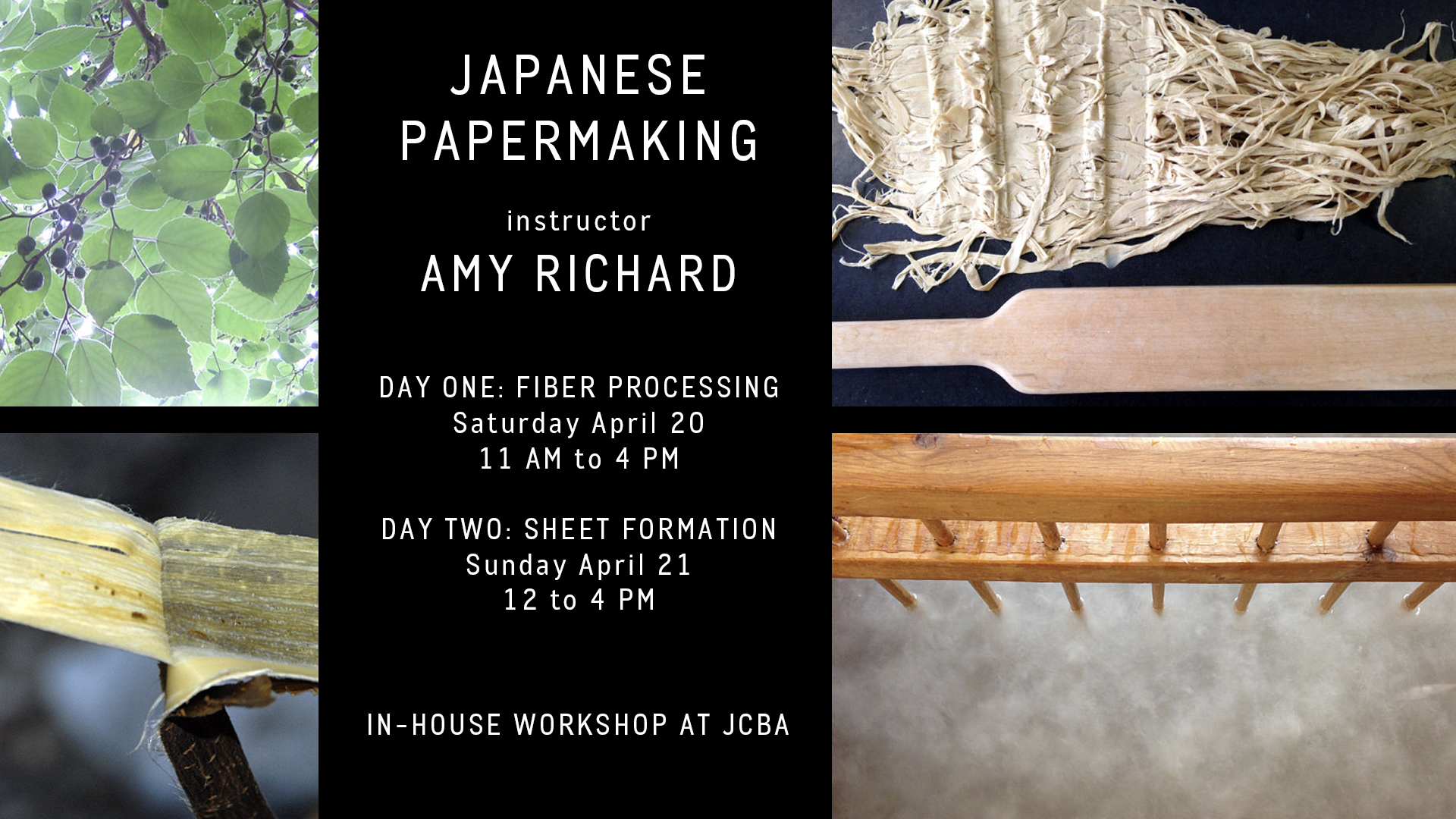The image is a high-quality advertisement flyer for an event titled "Japanese Papermaking" by instructor Amy Richard, hosted at JCBA. The central black text box with white print details the schedule: Day one, "Fiber Processing" on Saturday, April 20th from 11 a.m. to 4 p.m., and Day two, "Sheet Formation" on Sunday, April 21st from 12 to 4 p.m. 

The flyer is composed of four distinct photographs. In the top left corner, there is an image of a mulberry tree with leaves and berries, illuminated by sunlight. The top right features strips of natural oatmeal-colored paper and a long wooden paddle, suggestive of tools used in the papermaking process. The bottom left shows a close-up of plant fibers being pulled apart, revealing their intricate structure. Finally, the bottom right contains an image of a wooden oar or paddle, some string-like paper material in a paper-mache style, and a wooden railing leading into a misty background. These visual elements collectively emphasize the natural and artisanal aspects of the featured Japanese papermaking workshop.